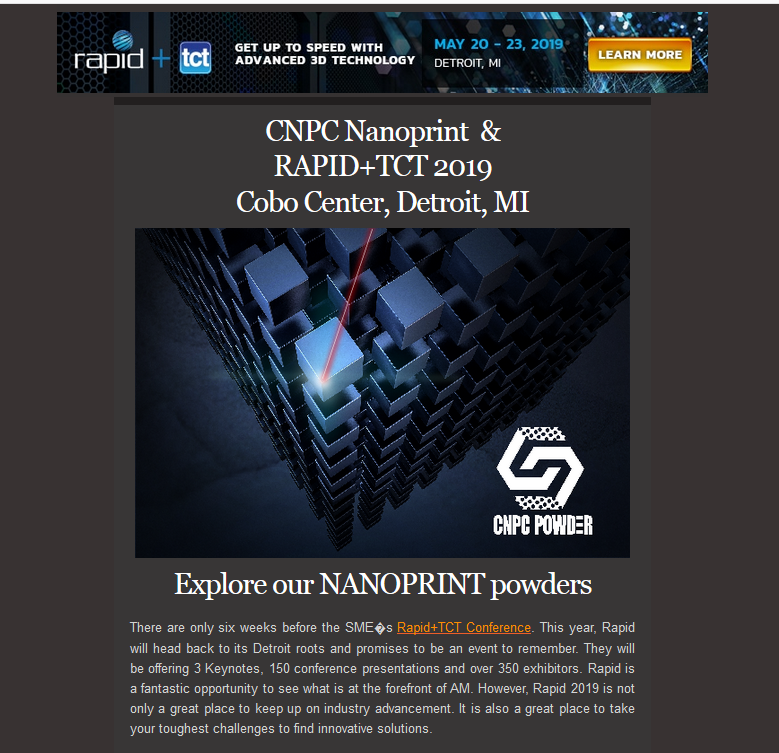**Detailed Caption:**

This image appears to be a promotional screenshot with a square format, suggesting it was extracted from a web page or a digital document. The background is a blend of brown and gray tones, providing a neutral backdrop for the other elements.

At the top of the image, there is a long rectangular banner stretching horizontally. This banner promotes the "RapidPlus TCT" event, with the tagline "Get up to speed with advanced 3D technology." The event dates are specified as May 20th through 23rd, 2019, and the location is Detroit, Michigan. On the right side of the banner, there is a prominent yellow button labeled "Learn More."

Below the banner, the background features white text mentioning "CNPC Nanoprint" and "RapidPlus TCT 2019" followed by "Cobalt Center Detroit Michigan," setting the stage for the event location and focus.

The central part of the image showcases a visually striking photo with a bluish-cobalt palette. It depicts several blue cubes seemingly levitating against the backdrop. A red laser beam is shown targeting one of the cubes, specifically hitting one of its corners, adding a dynamic and futuristic element to the scene.

Accompanying this visual, there is a caption that reads, "Explore our nanoprint powders," inviting viewers to delve into the featured technology. Additionally, the image contains the Nikon logo, along with a depiction of two metal C-shaped clamps positioned together, indicating the involvement of CNPC powder technology in the application.